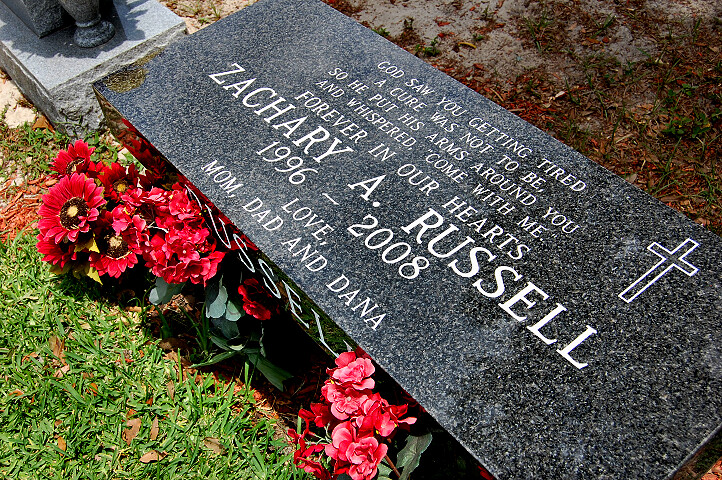This detailed photograph captures a somber scene at a cemetery, focusing on a dark-colored, rectangular headstone made of black and gray marble, positioned low to the ground. Engraved on the right side of the headstone is a cross, adding a touch of sanctity. The inscription reads: "God saw you getting tired, a cure was not to be, so he put his arms around you and whispered, 'Come with me,' forever in our hearts, Zachary A. Russell, 1996-2008. Love Mom, Dad, and Dana." Just in front of the headstone lie vibrant red zinnias, offering a contrast to the marble's dark tones. The green grass beneath the flowers and the brown earth provide a natural, serene backdrop, indicating that this peaceful scene was captured outdoors during the day. The photograph, taken at a slight angle from above, reflects care and reverence, immortalizing the memory of Zachary A. Russell.